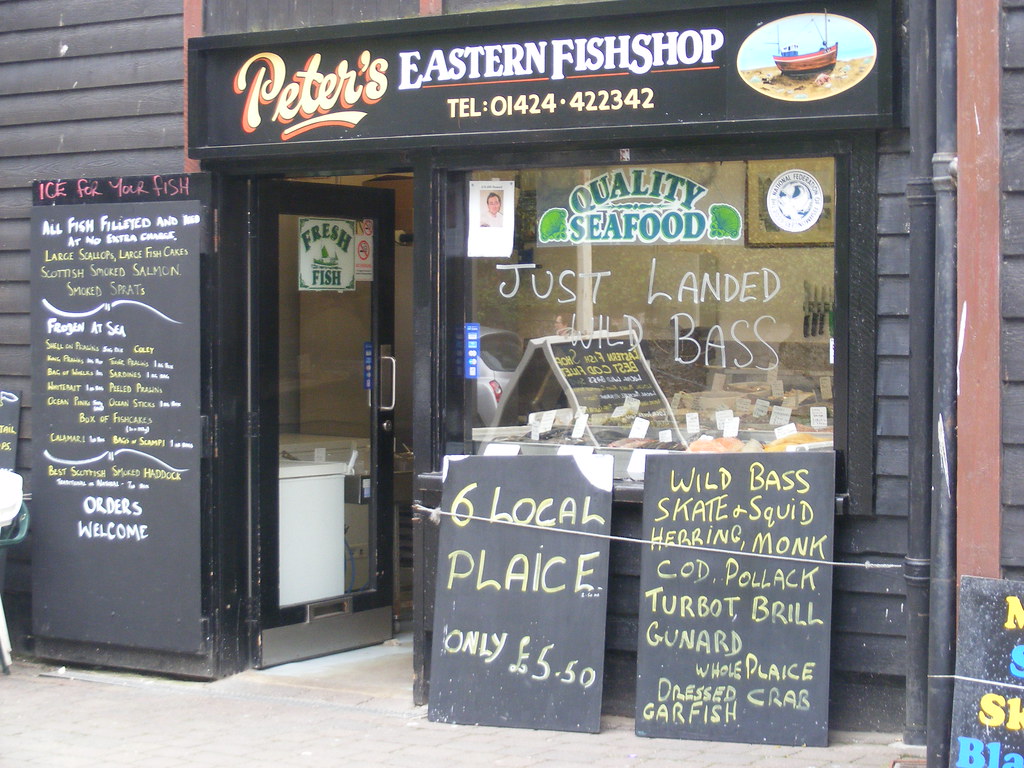In the full-color daytime photograph, an inviting fish shop in England is framed in a square format with no distinctive border or background. The shop's exterior is clad in blue wooden slats accented by off-red trim, exuding a charming rustic ambiance. Prominently displayed across the top is a black wooden sign featuring the name "Peter's" in bubbly cursive yellow text with an orange drop shadow, flanked by "Eastern Fish Shop" and a telephone number (01424-422342). An oval illustration of a boat on a beach further embellishes the sign.

To the left stands an open glass door, also painted black and adorned with a metal handle, inviting customers inside. The door sports a window with the words "Quality Food" inscribed on it. Adjacent to the door, a tall chalkboard menu lists today's offerings, while two smaller blackboards below the window advertise specials in cheerful yellow text.

Through the large window on the right, an enticing display of fresh seafood is visible, poised to tempt passersby. Bold white script on the glass announces "Just Landed Wild Bass," hinting at the day's fresh catch. The assortment includes wild bass, skate, squid, herring, monkfish, and grill, with prices such as "six local place, only £5.50" prominently highlighted. The storefront rests on a base of gray brick pavers, completing the picturesque scene of Peter's Eastern Fish Shop, where a variety of freshly caught fish promise a delectable culinary adventure.